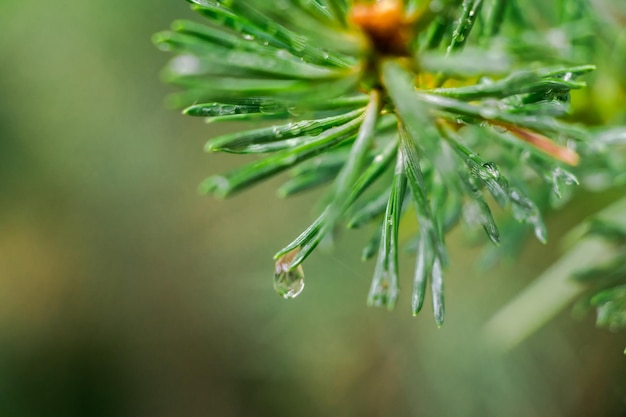This highly detailed macro photograph captures the very tip of a branch from an evergreen tree, likely a pine tree, thriving outdoors. The focus is on the intricate, spiky dark forest green pine needles adorned with dew drops. A closer inspection reveals a single large drop of water precariously hanging from one needle, just about to fall off. Evidence of the cold temperature is visible, as some of the water droplets appear to have frozen. Amidst the green needles, there are sections showing brown hints, specifically one brown needle off to the right and some brown at the center of the tip of the branch. The background is an artful blur of muted greens, yellows, and browns, accented with hints of red, lavender, and white, providing an abstract, textured backdrop that enhances the clear, sharp focus on the plant.